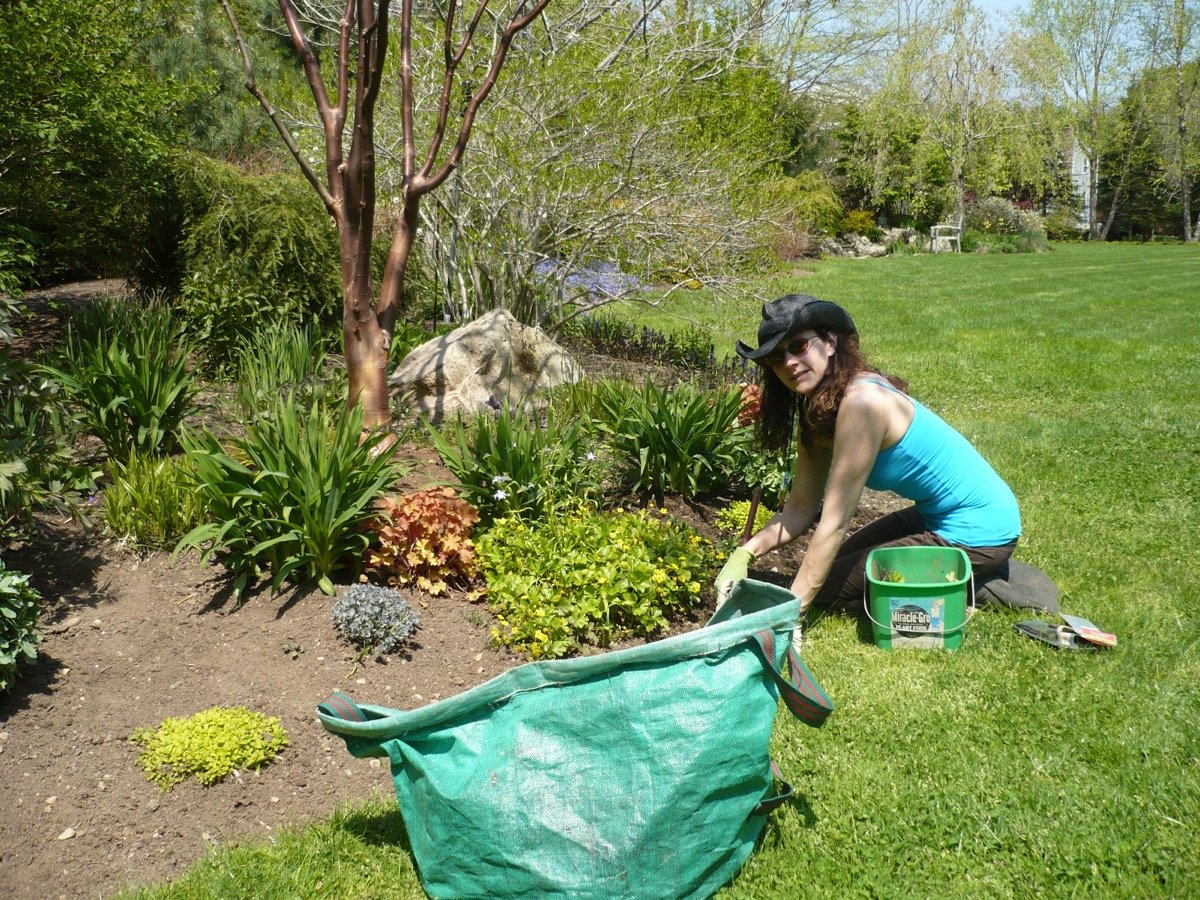The photograph captures a serene outdoor scene, featuring a young woman in her 20s or early 30s, engaged in gardening. She is kneeling on a well-maintained, expansive lawn, surrounded by an idyllic country setting. The garden plot she is tending is a circular area, adorned with flowering plants and a few bushes, with a tree placed centrally next to a large rock. The sky at the top right of the image is blue, adding to the tranquil ambiance.

The woman is looking towards the camera, wearing a black straw cowboy hat, sunglasses, a light blue tank top, brown pants, and black shoes. Her long dark brown hair cascades down, and she has a green glove on her right hand, which is actively digging into the dirt using a hand tool. Adjacent to her are gardening supplies: a green bucket labeled "Miracle-Gro," a white bag, and a teal vinyl bag. In the background, a white chair is visible across the lawn, along with a white house nestled in a more forested area, underlining the restful and picturesque countryside atmosphere.